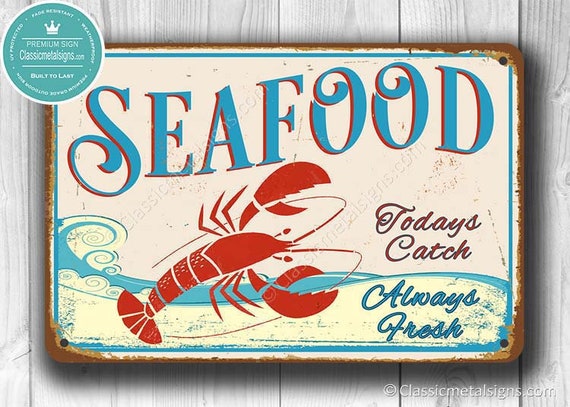Displayed on a weathered gray wall, the sign reads "Seafood" in large, stylized blue letters with red shadowing, dominating the top section. Below it, a vibrant red lobster is depicted against a backdrop of yellow sand and blue ocean waves, with its claws open as if bursting from the sea. To the right of the lobster, the words "Today's Catch" are written in cursive brown font, and beneath it, "Always Fresh" is boldly displayed in blue letters on the ocean waves. The sign has a white background with a blue border and an overall rustic appearance. A green seal in the top left corner features a crown and the text "Premium Sign, Built to Last," along with the watermark "classicmetalsigns.com" stamped below, suggesting its ironclad durability and origin. The sign exudes a classic seaside vibe, perfect for a seafood restaurant.